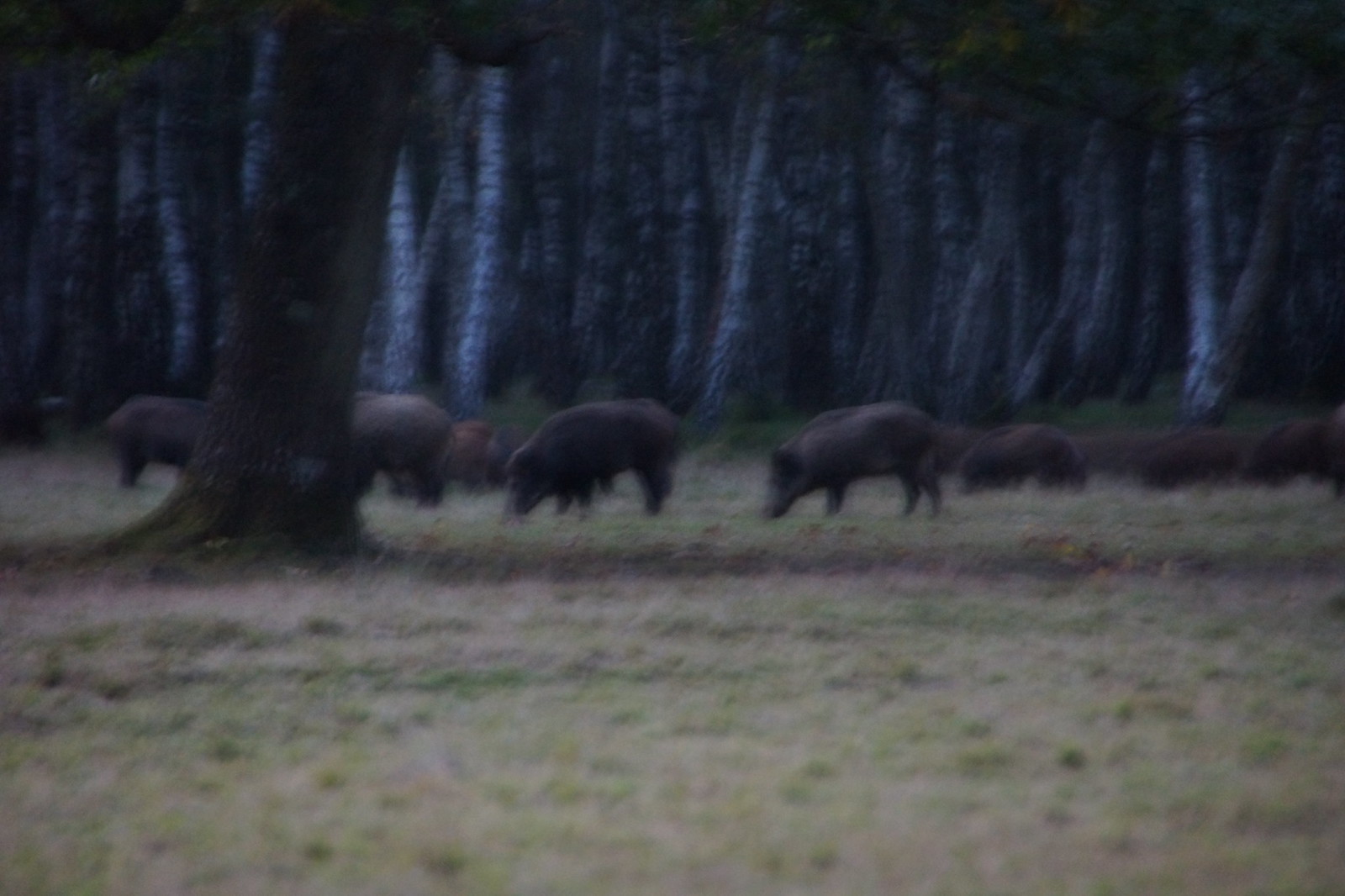The photograph, taken in landscape mode during the evening, is a blurry and out-of-focus image featuring wild boars in a trampled field. The wild boars, mostly chocolate brown and light brown, are grazing on the ground and are positioned horizontally across the center of the image, facing left. The field shows sections of light and dark green grass, tinged with brown and yellow due to trampling. In the foreground, there is a slanted tree with a large brown trunk. The background reveals a dense forest with a variety of tree trunks in shades of gray, white, chocolate brown, and light brown, accompanied by dark green foliage. Despite the poor image quality, the scene captures the wild boars in their natural habitat, surrounded by a thick wooded birch forest.